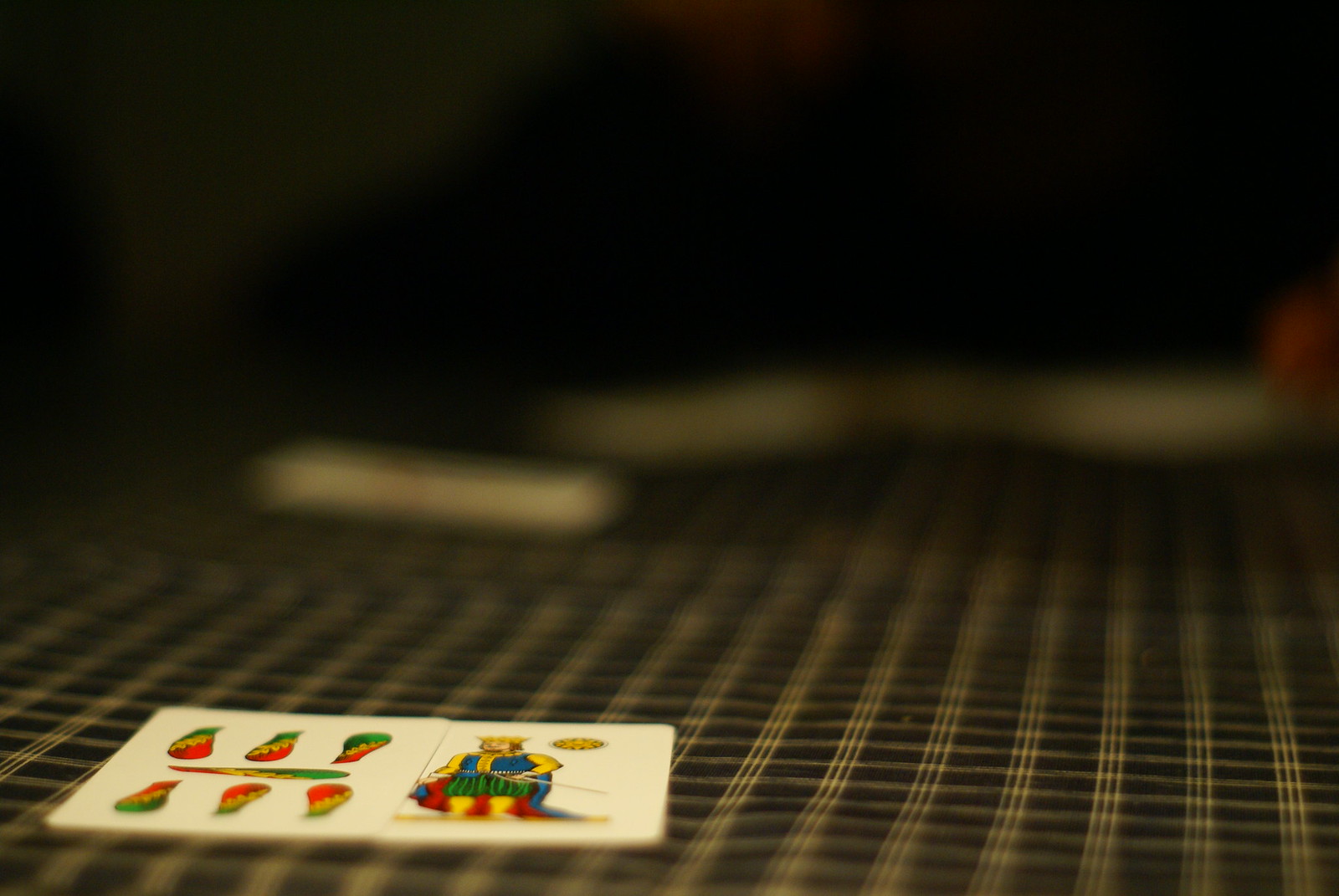This color photograph presents a partially out-of-focus image with a dark, blurry background. A figure, indistinct and surrounded by blurred white objects that may be cards or game pieces, appears seated behind a blue and white striped plaid tablecloth. In the bottom left corner of the image, two colorfully illustrated game cards slightly overlap on a white backdrop. 

On the first card, which features six jar-shaped objects, three at the top and three at the bottom, the top two are upright, while the third is upside down. Among the bottom three, the middle one is upright and the other two are upside down. A long feather-like figure occupies the center of this card. The objects on the top three have a green upper half, a central yellow leaf-like pattern, and a red lower half. The middle figure is colored inversely with a red top, the yellow pattern in the center, and green at the bottom. The bottom three objects mirror the top’s colors: red, yellow, and green respectively.

The second card depicts a regal figure, potentially a king, set against a white background. This character wears a yellow crown and shirt, a long blue vest-like garment, vibrant green, puffy pantaloon-style pants, and yellow stockings. The interior of the blue cape is a striking red. The king holds a large sword to the right and a blue object, likely part of the cape, in the left hand. A round yellow medallion adorns the top right corner of this card.